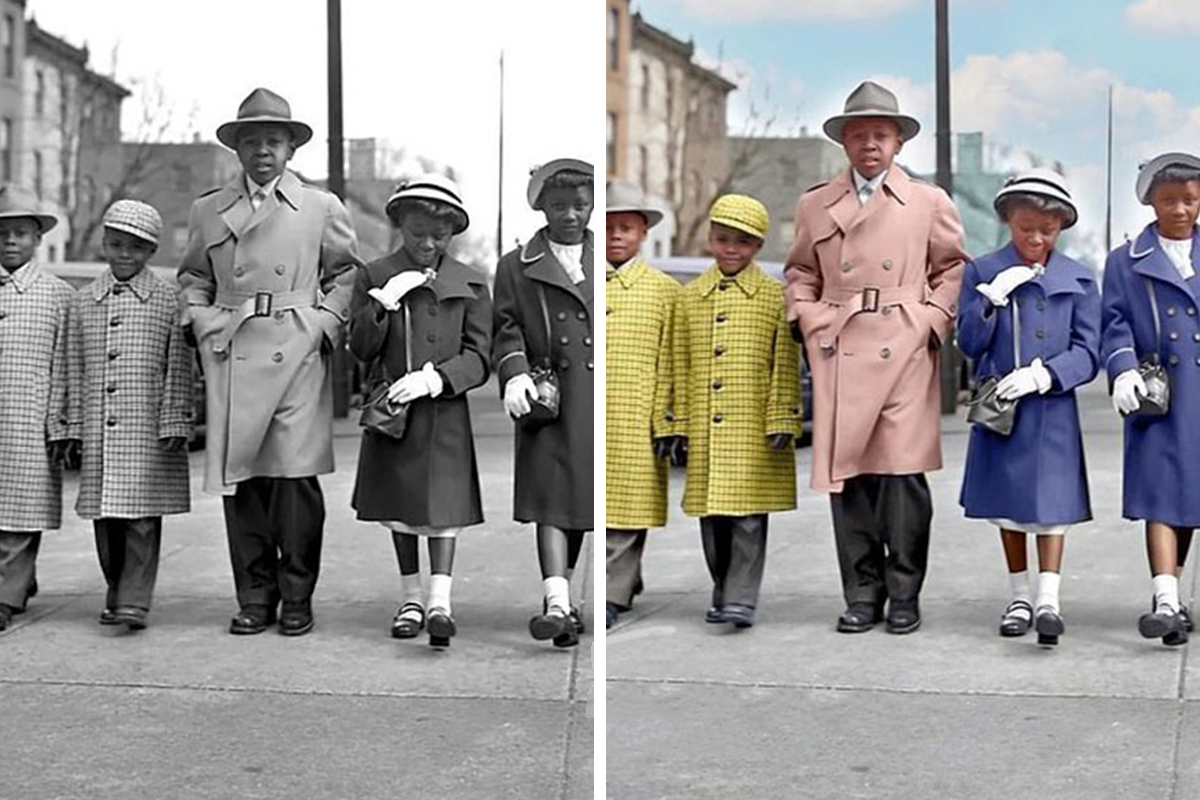The image showcases a remarkable coloration and restoration of a black-and-white photograph from the 1950s or early 1960s, featuring five African-American children. The original black-and-white image is displayed on the left, while the meticulously colorized version is on the right. In both versions, the children are arranged in a line, with two small boys on the left, a slightly taller boy in the center, and two young girls on the right.

In the colorized image, the transformation is vivid and brings out the details of their attire and surroundings. The boys on the left are adorned in bright yellow checkered jackets; one sports a yellow hat, while the other wears a gray fedora. The central figure, a slightly older boy, is dressed in a salmon-pink trench coat with a belt and visible buttons, paired with black slacks, black shoes, and a gray hat. His hands are casually tucked into his pockets as he gazes directly at the camera.

The two girls on the right are identically dressed in navy blue coats, white gloves, white socks, and black sandal shoes. They each carry a black handbag and wear white boater hats with black bands. The girl on the far right looks directly at the camera, while the other glances down at her handbag as they walk forward, adding a sense of motion to the scene. A clear, bright sky forms the serene backdrop of the colorized image, enhancing the overall vibrancy and historical charm of the composition.